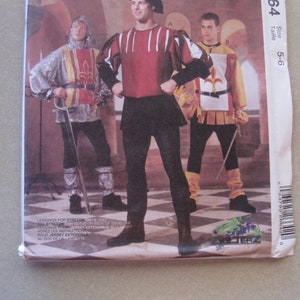This photograph captures a rectangular, plastic-wrapped package or box, resting on a gray table. The wrapper prominently displays a barcode on the bottom right and the numbers "64" and "5 through 6" printed on the right side. The front artwork illustrates a medieval-inspired scene featuring three young men, each dressed in period attire. 

The man on the left wears silvery chain mail, complete with a hood, and black tights accented with more chain mail at the bottoms. He is armed with a sword that he leans on, which extends from his hip to the ground. In the foreground stands a man proudly wearing a red and black shirt, a black skirt, and black leggings. He has a sword, is wearing black boots, and sports a confident smile. The man on the right is dressed in a yellow shirt with a white and red emblem, and black pants paired with yellow tights. He, too, wields a sword. The attire and accessories of all three lend the scene an air of medieval or renaissance nostalgia.